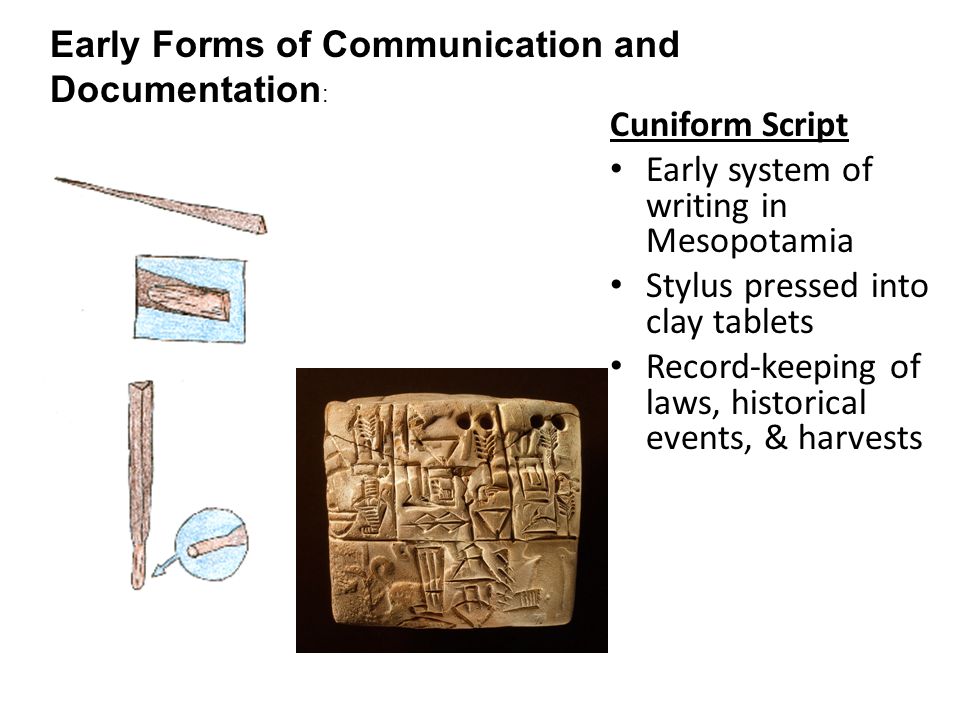The image is an educational depiction titled "Early Forms of Communication and Documentation," presented on a white background. The top-left corner features this title in black letters. The left side includes detailed illustrations of ancient writing tools, specifically a stylus used in Mesopotamia, shown in horizontal and vertical orientations with a close-up of its pointed tip. These tools were used to create cuneiform script by pressing into clay tablets, which are mentioned in the text under the heading "CUNEIFORM SCRIPT" on the top right. Below the heading, three bullet points describe cuneiform as an early system of writing in Mesopotamia, utilized for record-keeping of laws, historical events, and harvests. In the center bottom of the image, there is a photograph of a clay tablet inscribed with cuneiform symbols, displaying faint images, possibly of wheat and buildings, representing the types of records kept during that era.